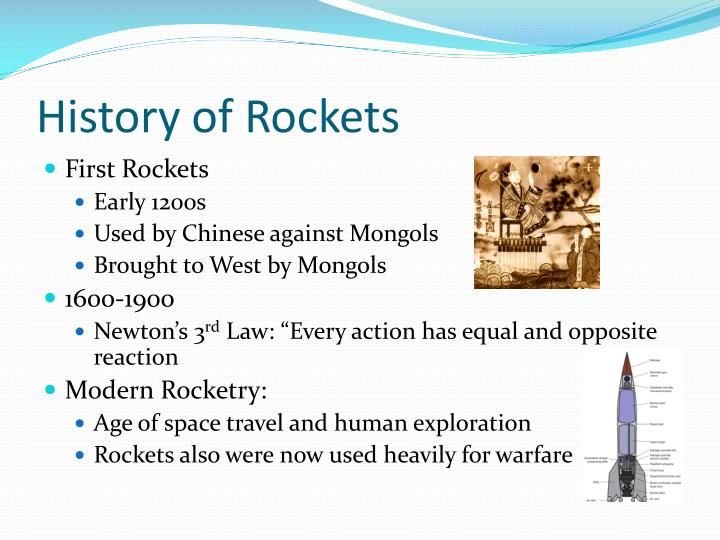The image features an educational PowerPoint slide with a white background and a blue wavy banner running across the top. The slide is titled "History of Rockets" in a blue font. Underneath the title, the information is structured with bullet points in aqua and sub-bullets in a darker blue. The slide is divided into three main sections: 

1. **First Rockets**:
   - **Early 1200s**: Used by Chinese against Mongols; brought to the West by Mongols.

2. **1600-1900**:
   - **Newton's Third Law**: Every action has equal and opposite reaction.

3. **Modern Rocketry**:
   - **Age of Space Travel and Human Exploration**: Rockets were now used heavily for warfare.

On the right side of the slide, there are two images. The upper image is a sepia-toned illustration that appears to depict ancient Chinese figures, possibly related to early rocketry. The lower image is a detailed, labeled diagram of a modern rocket with a gray body, purple accents, and a red tip.